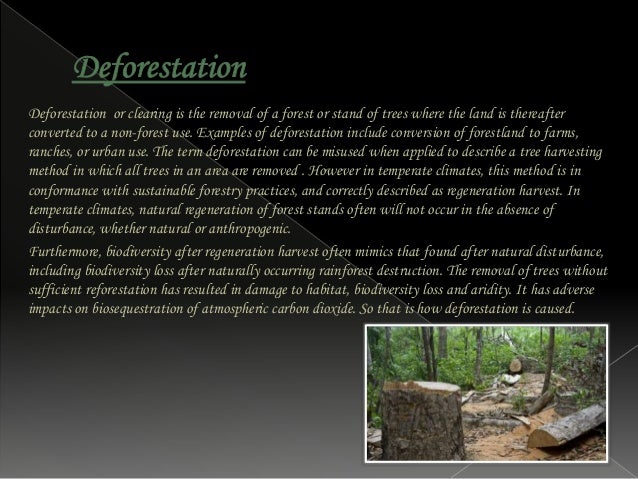The image features a PowerPoint slide with a background transitioning from black at the top to a lighter gray at the bottom. In the upper left corner, the word "Deforestation" is prominently displayed in underlined green letters. The main content consists of two detailed paragraphs in white font, discussing the concept of deforestation, defined as the removal of forests or stands of trees that are converted to non-forest uses such as farms, ranches, or urban areas. The text explains that the term "deforestation" can sometimes be misapplied when referring to tree harvesting methods. In temperate climates, the sustainable practice of regeneration harvest, where all trees in a specific area are removed to allow for natural or anthropogenic forest regeneration, is highlighted. The second paragraph delves deeper into the ecological impacts, noting that biodiversity after regeneration harvest often mirrors natural disturbances, including biodiversity loss, similar to naturally occurring rainforest destruction. It points out that insufficient reforestation can lead to habitat damage, biodiversity loss, increased aridity, and negatively affect the bio-sequestration of atmospheric carbon dioxide. In the bottom right corner, a small picture depicts a forest area with numerous trees cut down, showing trunks and tree debris scattered on the ground.